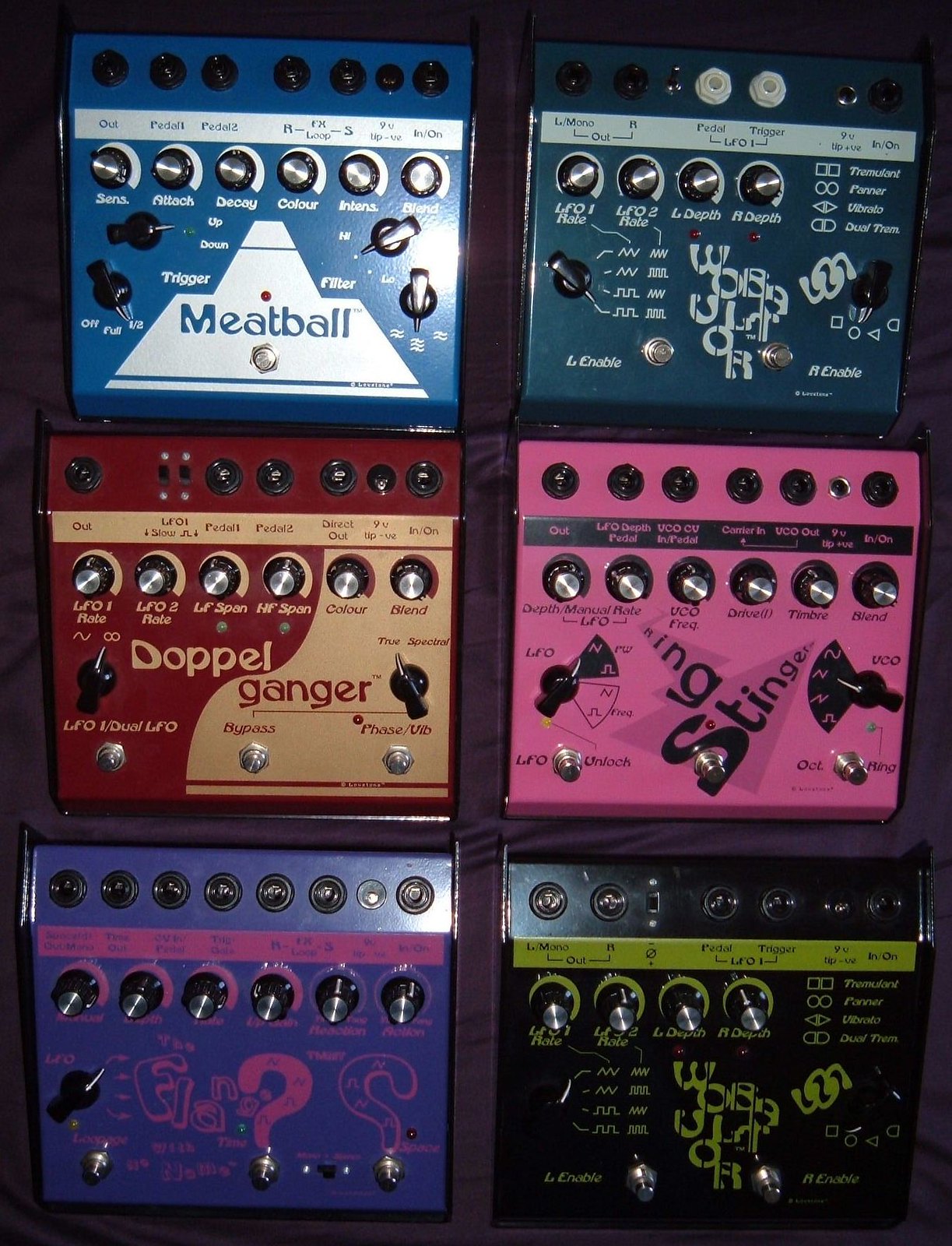The image is a detailed, portrait-shaped color photograph of six guitar pedals laid out on what appears to be a purple piece of fabric or bed sheet. The pedals are arranged in two columns with three rows, each featuring a distinct design and color. Starting from the top row, the left pedal is blue and labeled "Meatball," with numerous knobs and dials. The right pedal in the top row is a darker blue and is labeled "Wobbler," also featuring an array of knobs and buttons. In the middle row, the left pedal is red and beige and has "Doppelganger" written on it, while the right pedal is pink with the label "Stinger," both equipped with multiple control knobs. The bottom row has a purple pedal with some lime green markings, labeled "Flange," and the rightmost pedal is black with green patterns and fewer knobs, labeled again as "Wobbler." The pedals appear to be sitting against a dark brown or black wooden background and have a metallic and chrome finish on their various buttons and dials.